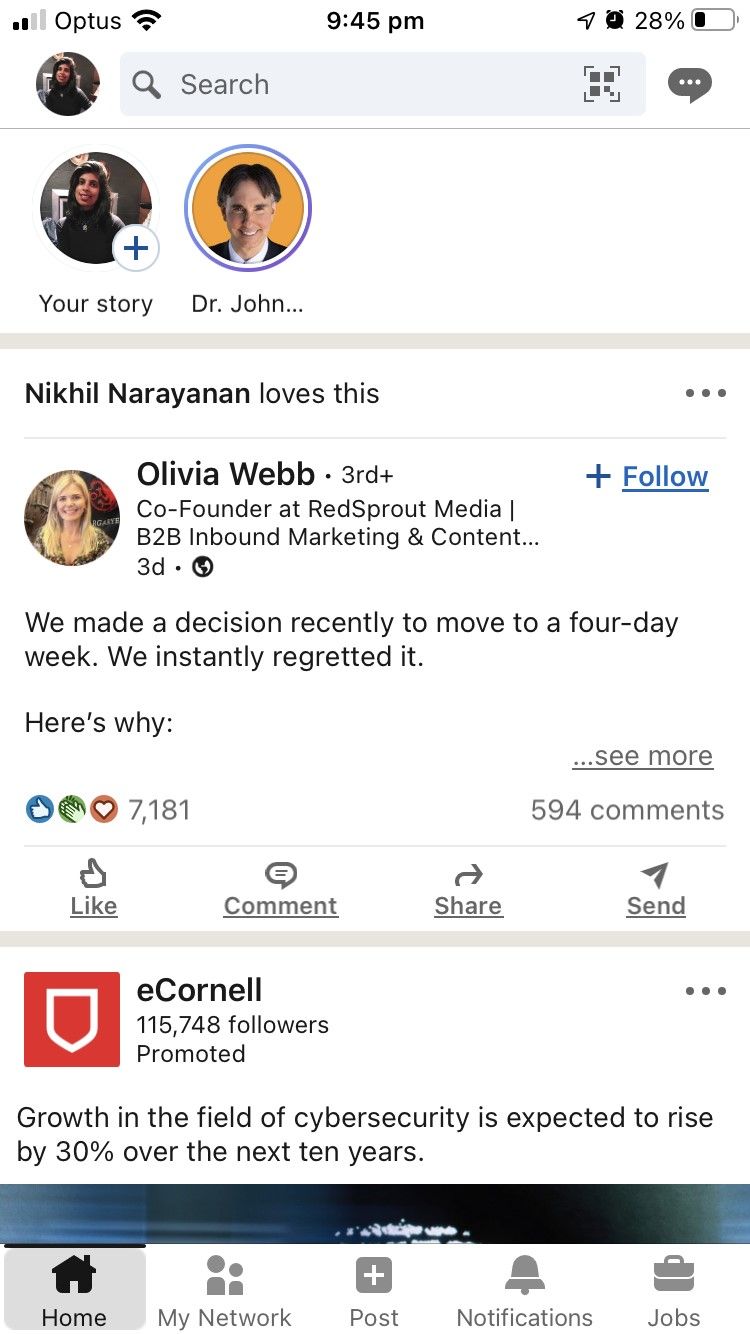This image is a screenshot of a social media page, potentially a networking platform. The top of the screen features a white status bar indicating the cell signal strength at two out of four bars, with Optus as the carrier. A Wi-Fi icon is displayed to the left, the time reads 9:45 p.m. in the center, and to the right, icons show that the alarm is set and the battery level is at 28%.

Beneath the status bar, there is a section displaying a profile picture of a woman with black hair, wearing a black jacket. Adjacent to the profile picture is a search bar, followed by options to add a story for this user, and a story from another user named Dr. John that is available to view.

Further down the page, there is a post by Olivia Webb. The content of Olivia's post revolves around recently transitioning to a four-day workweek and immediately regretting the decision.

Following Olivia's post, there is a promoted advertisement from eCornell. The ad highlights that growth in the field of cybersecurity is projected to increase by 30% over the next ten years.